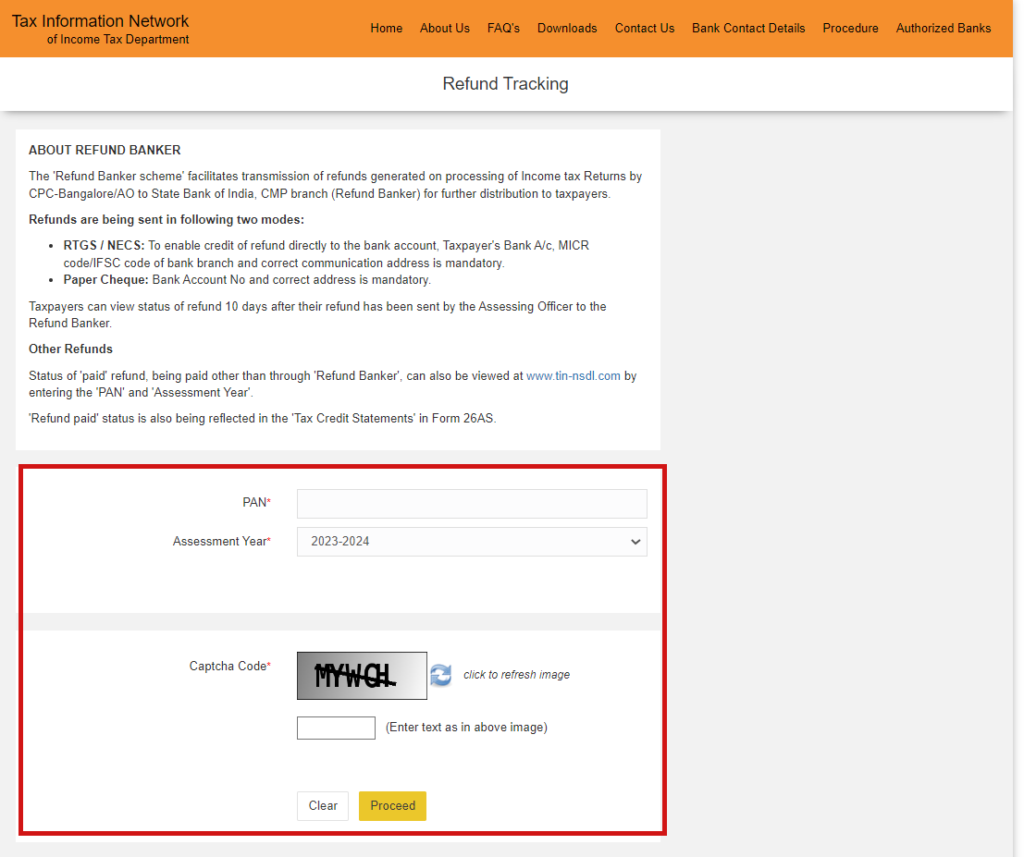The image displays a screenshot from a website related to the Tax Information Network, under the Income Tax Department. At the top, an orange banner prominently features the black text "Tax Information Network" on the left side, with "Income Tax Department" positioned beneath it. On the right side of the screen, a navigation menu lists several options, including: Home, About Us, FAQs, Downloads, Contact Us, Bank Contact Details, Procedure, and Authorized Banks.

Below the header, a white banner with the text "Refund Tracking" is centered. Further down, there is a gray background banner containing a white rectangle, which provides information under the heading "About Refund Banker." The text within explains that refunds are being sent through two modes: RTGS and ECS, and Paper Check. Additionally, it mentions that taxpayers can check the status of refunds 10 days after they have been dispatched by the assessing officer to the refund banker. It also notes that the status of other refunds, paid through methods other than the refund banker, can be viewed on the website by entering the PAN (Permanent Account Number) and assessment year.

Toward the bottom of the image, a red square outlines fields for user input. Inside, it prompts users to enter their PAN, marked with a red asterisk indicating that it is a required field. There is also a field for the assessment year, pre-populated with "2023-2024" and accompanied by a dropdown menu. Additionally, there is a prompt for users to enter a CAPTCHA code to proceed.